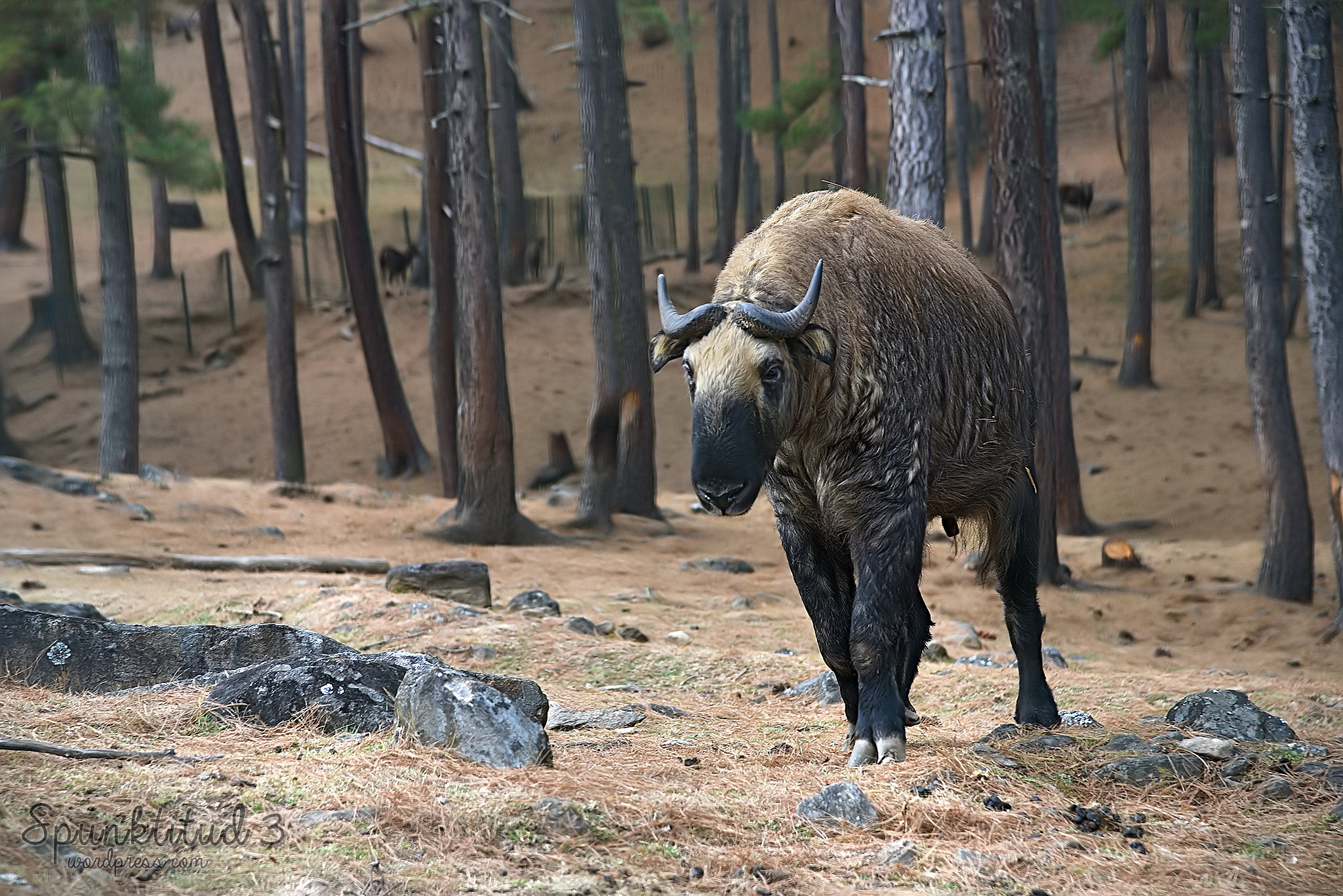The image depicts a desolate, burnt forest, with barren tree trunks reaching skywards and a hill in the background. The ground is a mixture of beige, straw-like grass and scattered rocks, suggesting a drought-stricken area. Dominating the foreground is an unusual animal that appears to be a hybrid of various species - it has the body and legs of a yak, a face resembling that of a moose, and horns akin to a water buffalo or ram. The animal's fur transitions from light brown on its upper body to dark brown or almost black on its legs, with gray hooves. Its expression seems forlorn as it stands in this sparse environment. To the left, a light, possibly black, fence ascends the hill, hinting at an enclosed space, potentially a zoo or animal reserve. Tucked at the bottom of the image is a watermark signature reading "SPUNKTITUDE 3" and a reference to a Wordpress page. This detailed scene combines elements suggesting both a naturally struggling ecosystem and human-managed wildlife area.